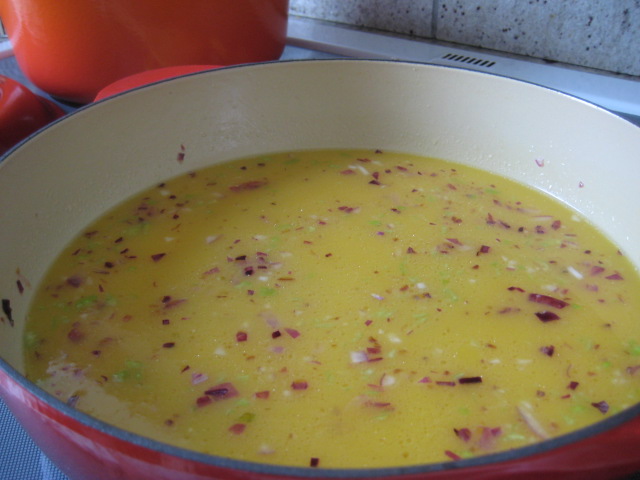The image depicts a rectangular photograph of a red, ceramic-lined pot standing on a silver surface, likely a stove. The pot, which is a wide shallow type, features a white interior with a black cast-iron rim. Inside the pot is a golden yellow, thick soup-like substance, resembling a corn soup or a sauce. This contents comes up two to three inches from the top of the pot. Floating in the mixture are fine, roughly chopped red onion flakes, small white flakes, and green sprigs, likely green onion and other herbs. In the background, there are two more red pots, with one pot being smaller and positioned to the left.